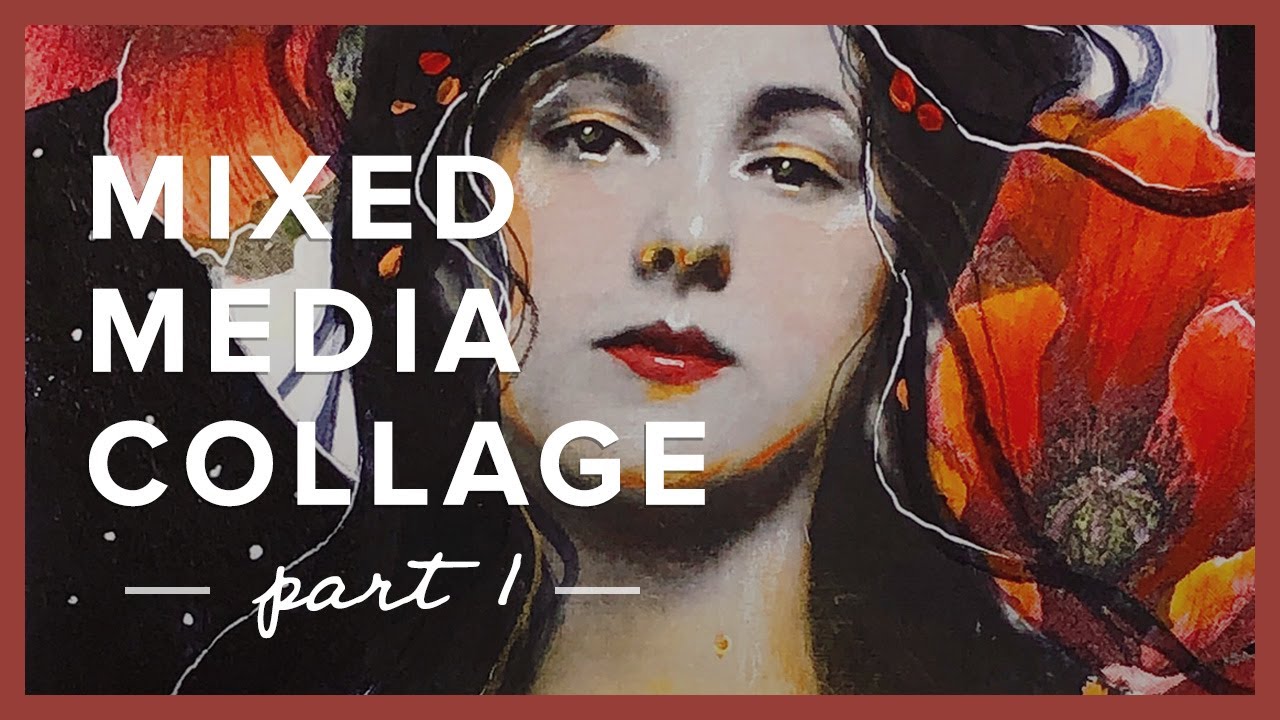The horizontally aligned rectangular image features a striking mixed media collage with a thick brown border. On the left side, white, all-caps text reads "MIXED MEDIA COLLAGE" in large block letters, followed by "PART ONE" flanked by dashed lines. This section is also left-aligned.

Dominating the center of the image is a detailed painting of a woman's face, visible from just above her mid-forehead down to her neck. Her skin is a grayish-white, almost porcelain-like, with subtle yellow highlights under her eyes, nose, lips, and chin. She wears dark red lipstick, which contrasts sharply with her black hair, containing white streaks. Her eyes are dark, accented with gold eyeshadow, and her black eyebrows add to her intense gaze.

Flanking her face are large flower petals. On the right, orangeish-brown petals with a darker center extend outwards, filling much of the space. Similarly colored petals are partly visible on the upper left side. The lower left side of the image features a mostly solid black background with scattered light gray spots.